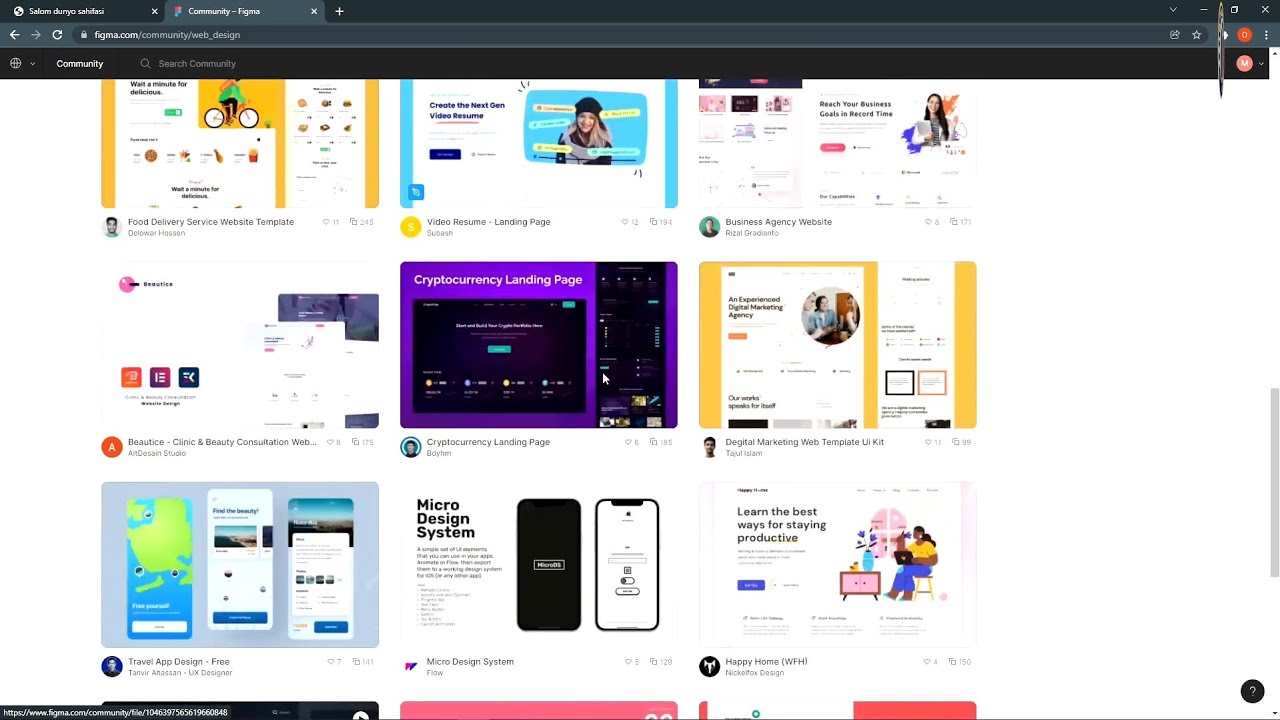The image is a detailed screenshot of a Figma website page. At the top of the page, a dark bluish gray header is prominently featured. In the top left corner of this header, a tab with a rounded bottom right corner displays a white globe icon to its left, followed by the white text "Salom Dunyo Sahifasi," and a white 'X' icon to the right. Adjacent to this is another tab, lighter bluish gray in color, adorned with an arrangement of colorful puzzle pieces forming an icon on its left, and the white text "Community-Figma" to its right, concluding with another white 'X' icon.

To the right of these tabs, within the darker bluish gray background, there is a white plus icon. Further along to the top right corner, four white icons are aligned: a downward pointing arrow, a minus sign, a maximize icon, and an 'X'.

Beneath this primary header lies a secondary lighter bluish gray header, which connects to the tabs. On its left, sequentially arranged, are a white left-pointing arrow, a light gray right-pointing arrow, a white refresh icon, and a long dark bluish gray URL bar with rounded ends. The URL bar features a white lock icon on the left, followed by the white text "Figma.com" and the light gray text "/community/web_design". On the far right end of the URL bar, there is a white square with rounded corners housing a white arcing arrow pointing to the right, followed by a white star icon.

The body of the page begins beneath these headers and features a black header with a white gridded globe icon in the top left corner, accompanied by a downward arrow, the white text "community," and a search bar to the right. The main content area of the page has a white background displaying various application information panes.